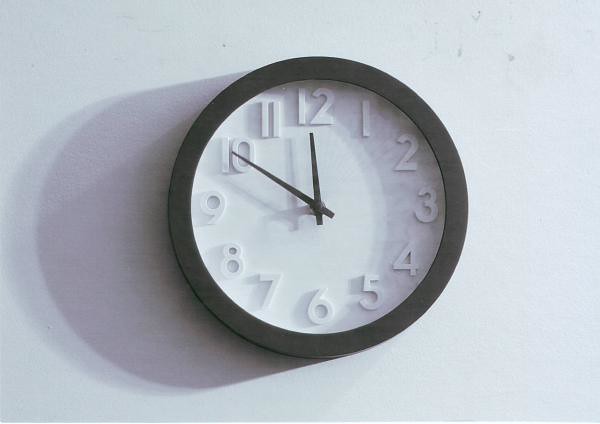The image depicts a clock prominently mounted on a wall. The clock features a minimalist design with a pristine white face, encased in a thick, bold black frame. The white clock face is accentuated by three-dimensional white Arabic numerals, which rise slightly from the surface, adding a subtle depth and ensuring the numerals are discernible despite the monochrome color scheme. The numerals range from one to twelve, indicating the hours. The clock's hands are sleek, with both an hour hand and a minute hand, currently showing the time as 11:50, suggesting that it's about to strike midnight.